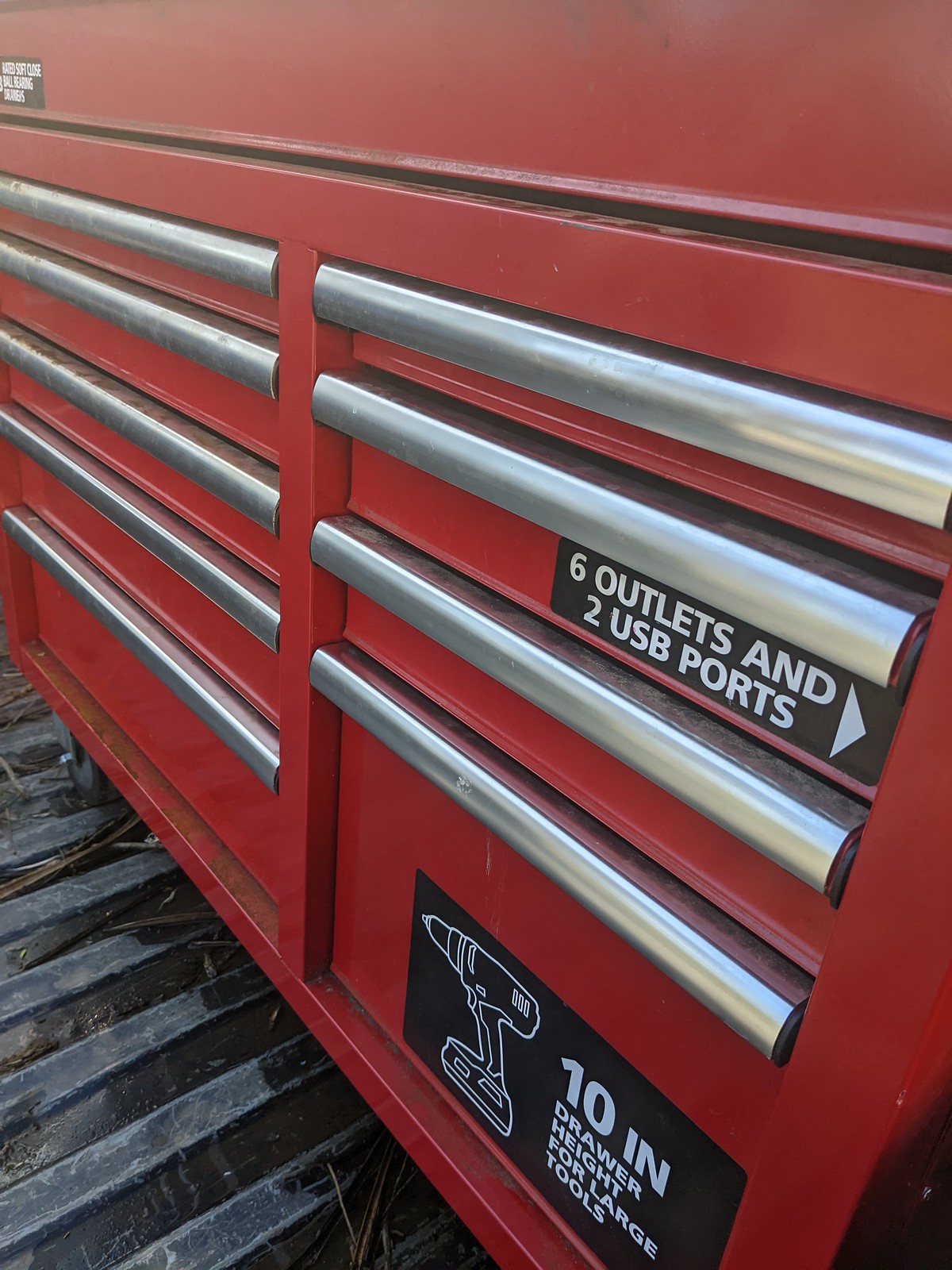The image is a vertical, realistic photograph dominated by a large red metal tool case that spans from the bottom right corner up towards the middle left side of the frame. The toolbox, made of red metal, features multiple drawers with stainless steel handles. There are five drawers on the left and four on the right, prominently positioned at the front. The ground or flooring in front of the toolbox is black and grooved, possibly resembling the floor of a truck. Two black signs affixed to the right side extend additional detail: the upper sign, with white text, reads "six outlets and two USB ports" with an arrow pointing to the right, while the lower sign showcases the outline of a hand drill and states "10-inch drawer height for large tools." The overall texture and meticulous details suggest the tool case is intended for housing various tools, providing both storage and power outlets.